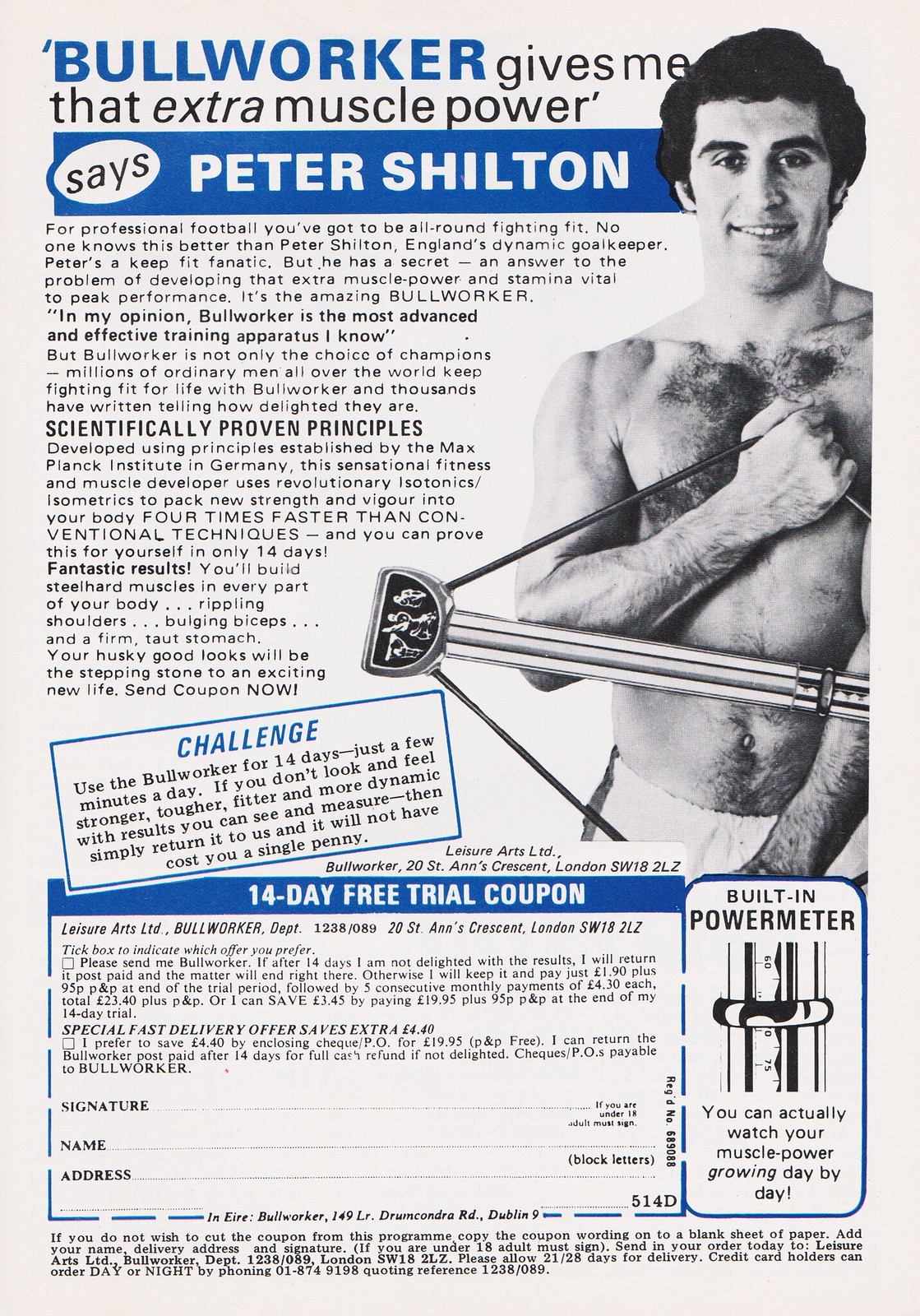This image, taken from an old magazine, features an advertisement for the Bull Worker exercise equipment. At the top of the portrait-style page, the brand "Bull Worker" is written in bold blue letters, followed by the black text "gives me that extra muscle power." A blue bar containing the black text "Says" and white text "Peter Shilton" follows.

Centrally positioned on the right is a photograph of a shirtless man, identified as Peter Shilton, England's renowned goalkeeper. He is depicted mid-exercise, pulling a Bull Worker device—a piece of exercise equipment that resembles a bow and arrow—demonstrating its use with one hand pulling upward and the other downward. He is wearing white shorts.

To the left of the image, paragraphs of text explain the scientifically proven principles of the Bull Worker and its benefits for muscle power, citing its efficacy endorsed by Shilton. A detailed challenge is outlined in a blue-bordered box in the middle of the page, urging readers to use the Bull Worker for 14 days. The text promises that just a few minutes of daily use will visibly improve strength, toughness, fitness, and dynamism. If unsatisfied, users can return the product without any cost.

At the bottom of the ad, a 14-day free trial coupon is available for readers to fill out and mail. The coupon includes fields for a signature, name, and address, framed by a blue bar with white text reading "14 day free trial coupon." Adjacent to the coupon, a logo and accompanying text highlight a built-in power meter feature, which allows users to track their muscle growth daily.